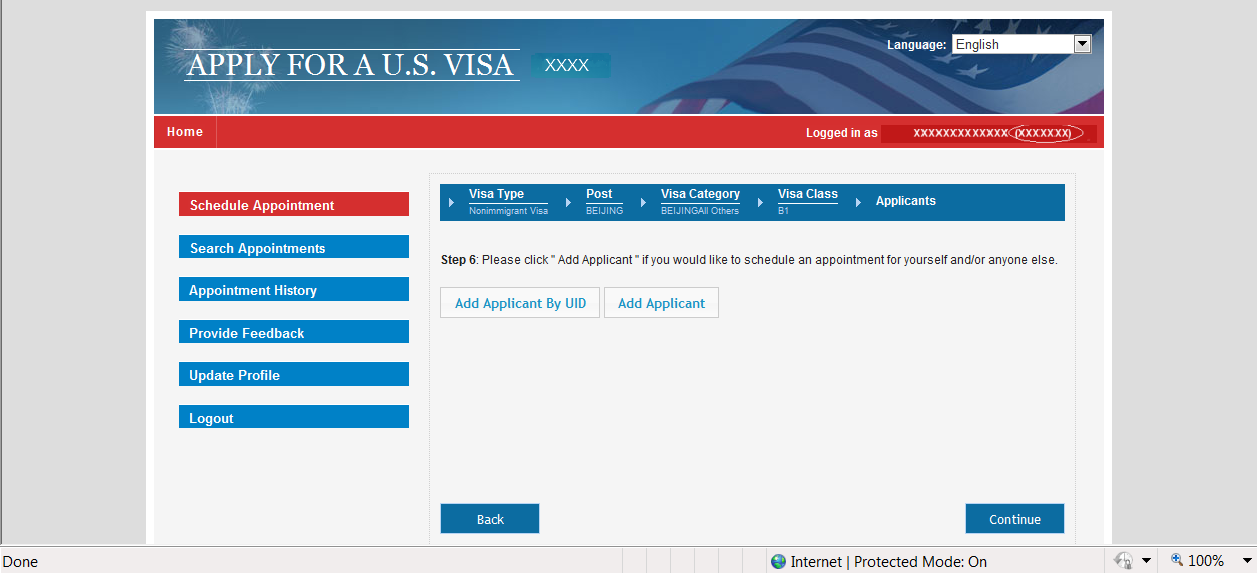**Detailed Caption for Screenshot of Visa Application Website Interface:**

The screenshot showcases a zoomed-in view of a visa application website, framed by a gray border along its outer edges. At the bottom taskbar, there are status indicators: "Done" appears in the bottom left, while "Internet Protected Mode: On" is centered. The bottom right displays a zoom control feature set to "100%" with a drop-down menu for adjustments.

At the top of the web page, a blue sky background adorned with fireworks on the left and an American flag on the right sets a patriotic theme. In the upper right corner, there's a drop-down menu labeled "Language: English." 

On the upper left, the text "Apply for a U.S. Visa" is prominently displayed, followed by a red banner below it stating "Apply for a US Visa." Beneath the red banner, there is a navigation menu that reads "Home," "Logged in as," alongside a user identifier symbolized by "XXXXXXX."

Further down, the interface shows a red button labeled "Schedule Appointment," followed by a series of blue links: "Search Appointments," "Appointment History," "Provide Feedback," "Update Profile," and "Log Out."

On the right side, the user is provided with visa-specific options and instructions, mentioning "Visa Type: Non-Immigrant Visa," "Post: Beijing," "Visa Category: Beijing Others," and "Visa Class: B1." A detailed step-by-step instruction section follows: "Step 6: Please click 'Add Applicant' if you would like to schedule an appointment for yourself or anyone else," with options to "Add Applicant by UID" or "Add Applicant General." At the bottom, navigation buttons include "Back" and "Continue."